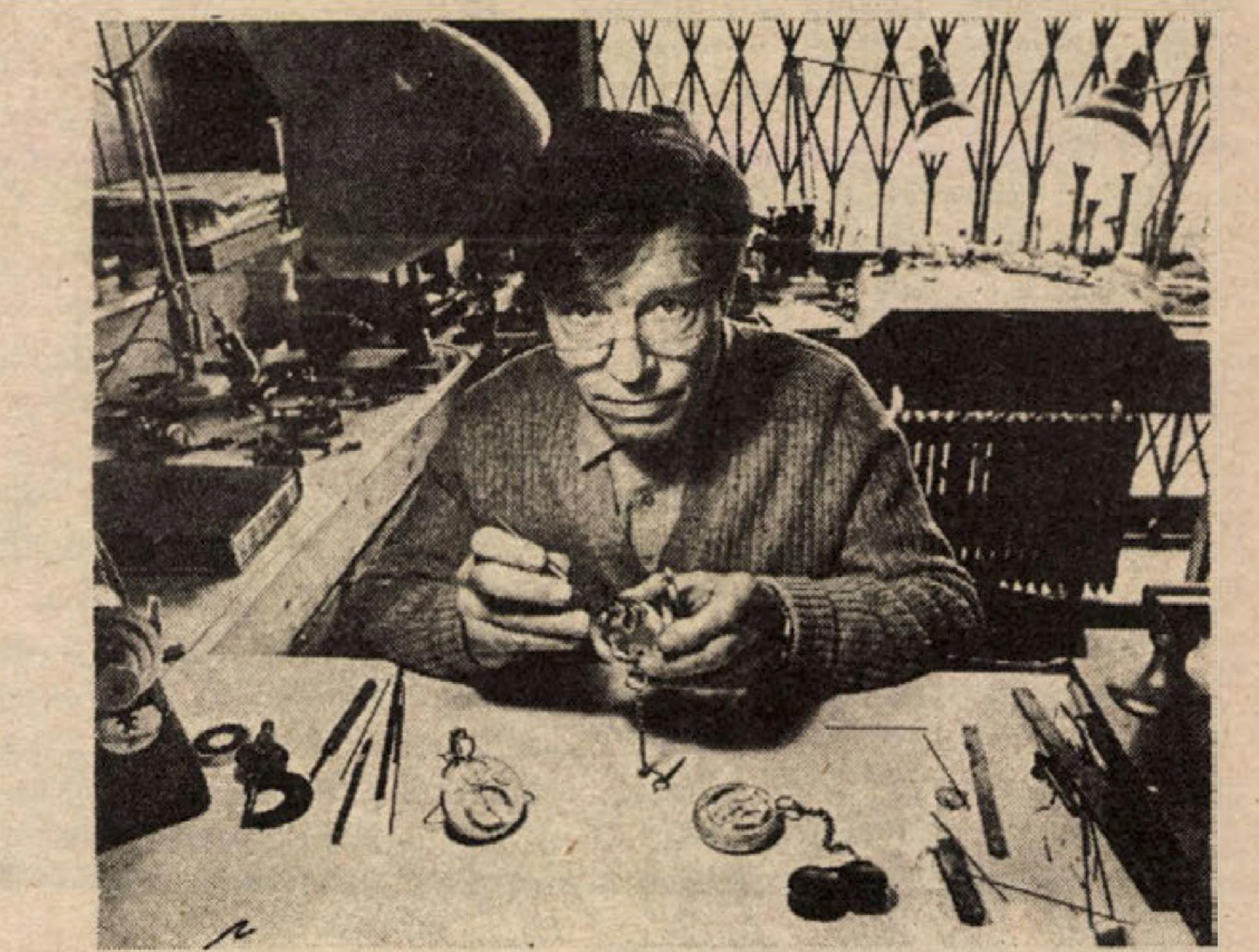A black and white photograph, reminiscent of a newspaper clipping, captures a man with dark hair and glasses perched low on his nose, seated at a cluttered and messy workbench. He wears a buttoned-up shirt underneath a cardigan sweater and is engaged in the intricate repair of a pocket watch, holding a tool up to the open device. The man's workspace, presumably an at-home or simple shop workshop, is filled with tiny screwdrivers, pocket watches, and other fine tools scattered across a wraparound countertop that extends the length of the wall. Behind him, the disarray continues with numerous tools and a distinctive accordion-style metal grate covering what is likely a window. Two lamps illuminate his workstation. The man is looking up from his meticulous work, with a slight smile, directly at the camera.